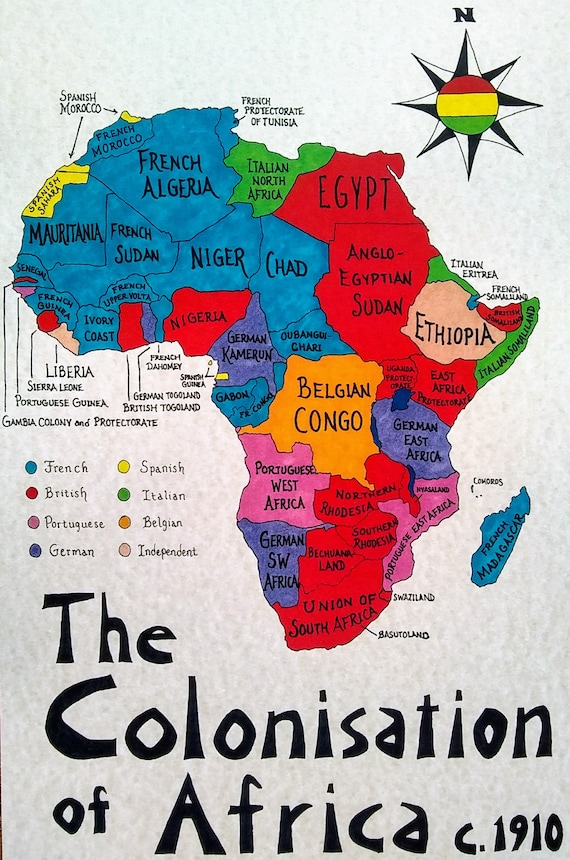The poster, titled "The Colonization of Africa, circa 1910," displays a detailed map of Africa during the colonial era, segmented into various countries and colored according to their respective colonial rulers. The rectangle-shaped poster, presented in portrait view, features a prominent star compass in the top right corner with a north arrow pointing upward, embellished with the colors of the Ethiopian flag—red, yellow, and green.

The map divides the continent into regions controlled by different empires, coded by color for easy identification. French colonies, all shaded in blue, include Tunisia, Algeria, Morocco, Mauritania, French Sudan, Niger, Chad, Ivory Coast, French Upper Volta, French Guinea, and Senegal. Spanish territories, marked in green, encompass Spanish Sahara and Spanish Guinea. The Italian-controlled areas, also in green, cover Italian North Africa, Italian Eritrea, and Italian Somaliland. British colonies, shaded in red, consist of Egypt, Anglo-Egyptian Sudan, East Africa Protectorate, British Somaliland, and several southern regions including Northern Rhodesia, Southern Rhodesia, Bechuanaland, and the Union of South Africa, along with Aro-Seng Basutoland and Swaziland.

German colonial territories, highlighted in dark blue, include German Cameroon, German East Africa, and German South West Africa. The Portuguese regions, depicted in pink, include Portuguese West Africa and Portuguese East Africa. Belgian Congo is marked in a light green-yellow shade, and areas designated as independent are colored in a distinct peach hue.

Additional details include a key indicating the color code for each colonial power, positioned to the left of the map. This key clarifies that blue represents French colonies, red for British, pink for Portuguese, dark blue for German, green for Italian, light green for Belgian, and a creamy color for independent regions. 

At the very bottom of the poster, the title "The Colonization of Africa, circa 1910" is prominently displayed, encapsulating the historical essence of the depicted colonial divisions.